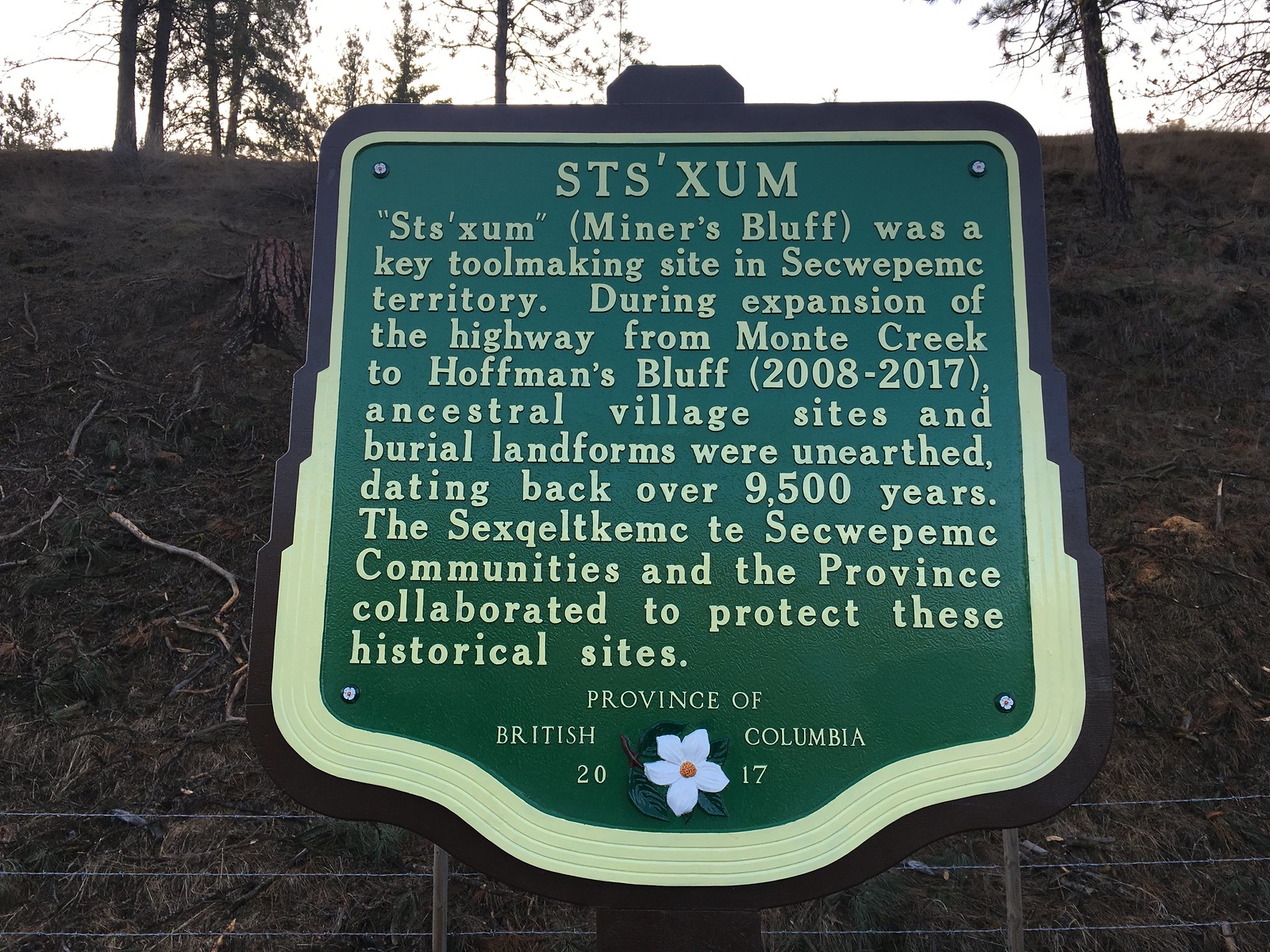The image showcases a green metal sign, mounted on wooden posts, positioned above a stone or tiled path, set against the backdrop of a forest. The sign reads "STSXUM" at the top and the same word is noted just below. In parentheses, it includes "Miner's Bluff," identifying the location as a significant tool-making site within the Secwépemc territory. The detailed text explains that, during the highway expansion from Monte Creek to Hoffman's Bluff between 2008 and 2017, ancestral village sites and burial landforms were discovered, dating back over 9,500 years. Mentioning the Sekwempik and Secwépemc communities, it highlights their collaboration with the province to protect these historical sites. At the bottom, the sign is marked with "Province of British Columbia, 2017," symmetrically flanked by a white dogwood flower separating the two parts of the year.